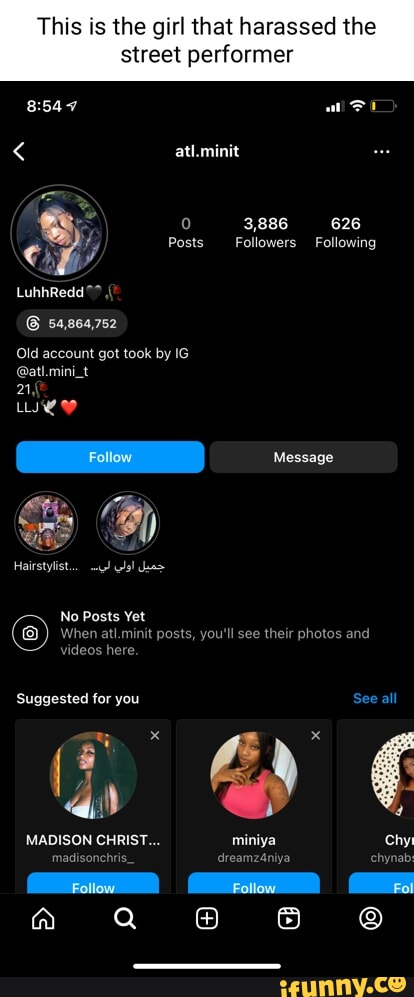A smartphone screenshot shows the profile of an Instagram user named "L-U-H-H-R-E-D-D," who is described by the caption at the top as "the girl that harassed a street performer." The time displayed on the screenshot is 8:54. The profile picture features a heavyset Black woman. The account statistics are shown as "ZERO POSTS," "3,886 followers," and "626 following." Additionally, a note under the username reads, "this old account got took by IG." Below this information, there is a blue "Follow" button and a gray "Message" button. The text also indicates that there are no posts yet with the message: "When ATL.MINIT posts, you'll see their photos and videos here." At the bottom, there is a "SUGGESTED FOR YOU" section featuring three additional accounts, each with a profile picture and a follow button.